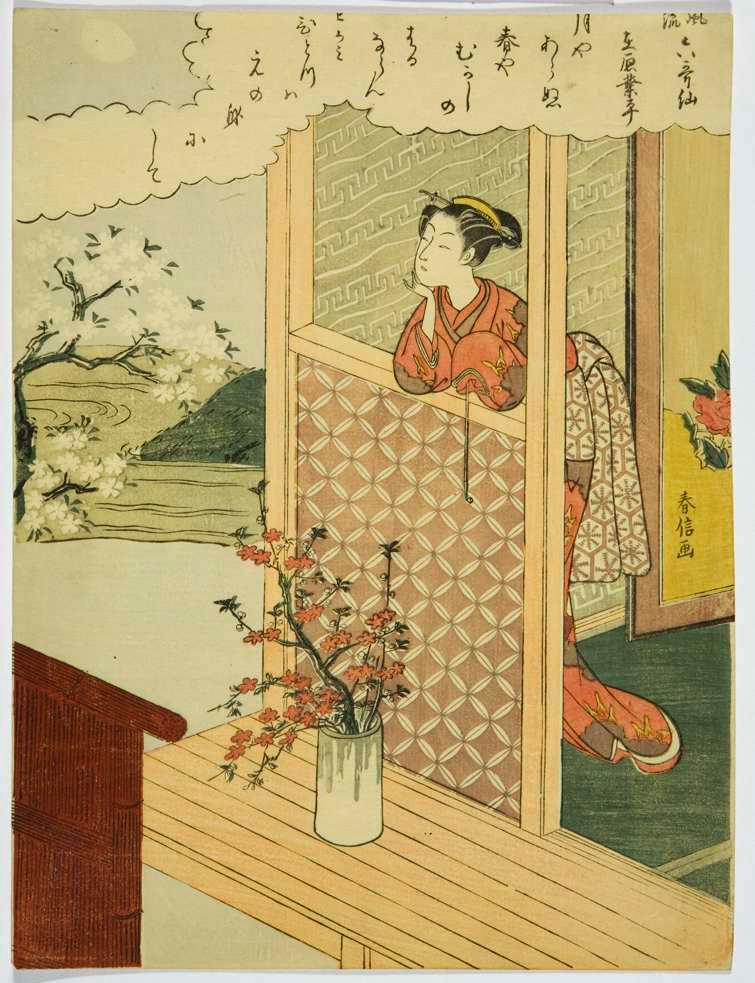The image depicts a piece of Asian animation style artwork with a richly detailed scene. In the background on the left-hand side, there's a gradation of light gray to darker tan hues forming the sky, and in the top left, a round, yellow circle represents either the sun or the moon. A large cloud stretches from left to right and is filled with various types of Asian writing, resembling a collection of phrases. Below this cloud, the landscape features a hill with a bent tree on the left, from which several small leaves are flying off. To the right of the tree is an open-air room with a light tan window frame, where a woman dressed in an orange kimono, styled as a geisha, leans her elbows on the window sill in a contemplative pose, her hand resting on her chin. She has her hair tied back with a yellow hair ornament. The wall behind her is light pink with white diamond shapes, and at the bottom, a yellow trim stands out. The room has a green carpet, and outside on the light tan wooden porch, there's a pot of orange flowers adding a pop of color to the scene.